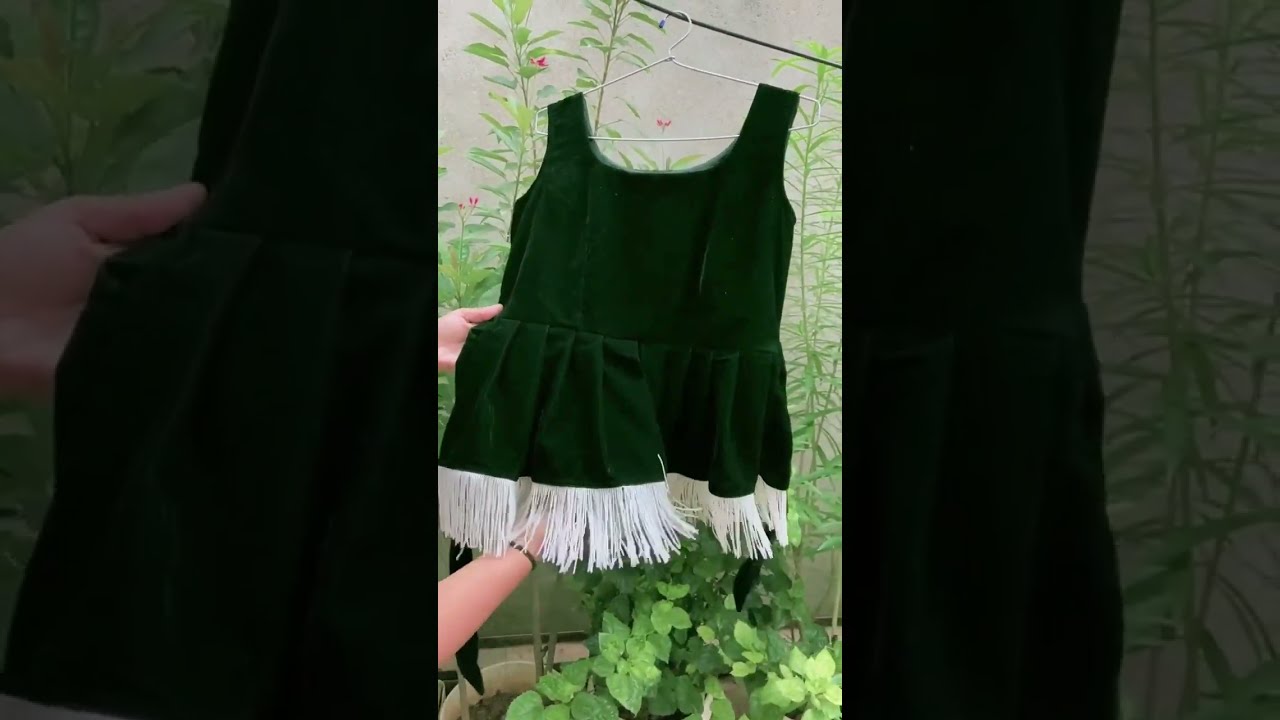The photograph features a small, dark green child's dress, likely made of velvet, adorned with white fringe or tassels along its bottom edge. The dress, which includes a pleated waist, hangs from a white wire hanger suspended on a clothesline. Two Caucasian hands are visible, one holding the dress at the waist and the other underneath the fringe, displaying the garment. The scene appears to be set in what could be a greenhouse or a garden, with a foggy backdrop featuring leafy green plants and some fern-like foliage with yellow-orange buds. The image itself seems to be taken with a cell phone and is formatted with broad darkened strips on either side, showing closer, darkened sections of the dress, hands, and some background foliage. The overall setting includes a gray wall, possibly adorned with painted plants, and real ivy climbing upward, emphasizing the lush, botanical feel.